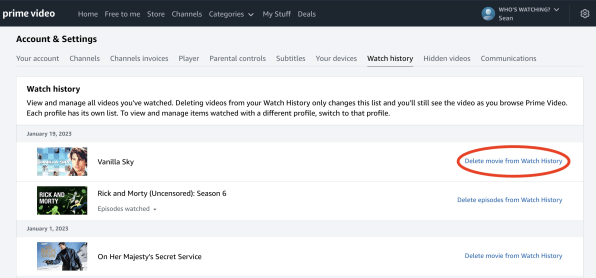The image is a detailed screenshot of a specific section of the Prime Video website. At the very top, a black navigation bar is visible, with "Prime Video" written on the left-hand side. Centrally aligned on this bar are several options: "Home," "Free2Me," "Store," "Channels," "Categories," "My Stuff," and "Deals." On the far right side, there is a drop-down menu labeled "Who's Watching?" accompanied by a blue person icon. Below this icon, the name "Sean" is displayed. The far corner of the bar features a settings wheel icon.

Beneath the black bar lies a light gray section titled "Account and Settings." This section includes a list of options: "Your Account," "Channels," "Channels Invoices," "Player," "Parental Controls," "Subtitles," "Your Devices," "Watch History" (which is currently selected), "Hidden Videos," and "Communications." 

Following this is a series of lighter white blocks. The first block is labeled "Watch History" and provides instructions: "View and manage all videos you've watched. Deleting videos from your watch history only changes this list. You’ll still see the video as you browse Prime Video. Each profile has its own list. To view and manage items watched with a different profile, switch to that profile."

Under the instructions, the date "January 19, 2023" appears, followed by icons for two videos: "Vanilla Sky" and "Rick and Morty Uncensored, Season 6, Episodes Watched." Further down, the date "January 1, 2023" is listed along with an icon for "On Her Majesty's Secret Service." To the right of each video entry, there is blue text that reads "Delete Movie from Watch History." Notably, the delete option next to "Vanilla Sky" is circled in red.